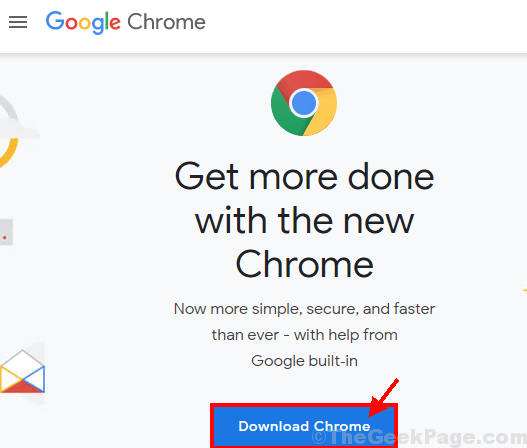The screenshot displays a Google Chrome promotional webpage viewed on a desktop using the Google Chrome browser. At the top of the image, the Google Chrome browser window is visible with the browser's "three-line" menu icon. The main content of the webpage is presented on a gray background.

At the top of the page, the Google Chrome logo is prominently displayed. Directly beneath the logo, there is a headline in black text stating, "Get more done with the new Chrome." Following this, a subheadline reads, "Now more simple, secure, and faster than ever – with help from Google built-in."

Below this text, a large blue rectangular button with white text commands immediate attention, urging users to "Download Chrome." The button is accented with a red trim and a red arrow pointing to it.

A grayed-out copyright notice for "The Geek Page" is faintly visible near the bottom of the screenshot. On the left side of the image, there are a few small, indistinct icons; one of these icons, located at the bottom, resembles an open envelope.